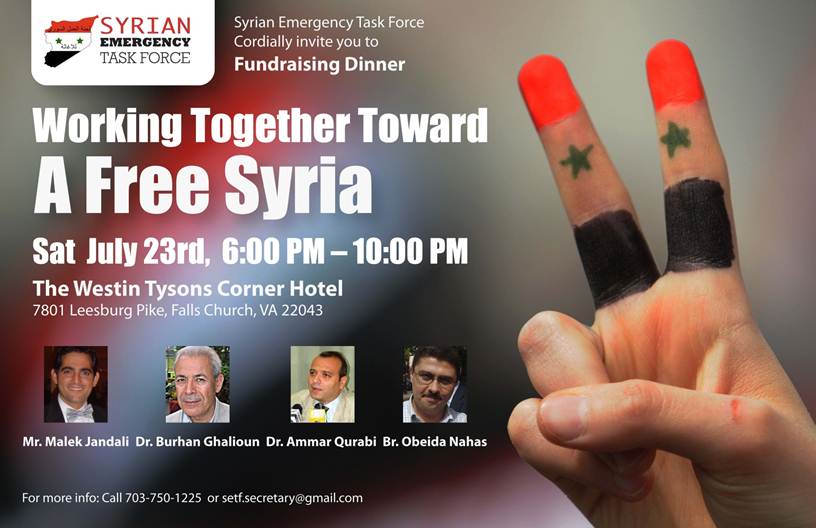This horizontal rectangular advertisement is for a fundraising dinner organized by the Syrian Emergency Task Force. The large right portion of the image prominently features a human hand displaying a peace sign with the Syrian flag painted on the two upraised fingers. The tips of the fingers are red, followed by segments featuring a green star, and black, representing the Syrian flag. In the top left corner is the Syrian Emergency Task Force's logo, which depicts a stylized map of Syria adorned with the colors of the Syrian flag—red, white, and black, with two green stars.

The main message in bold text reads, “Working together towards a free Syria,” with smaller text below detailing the event date and location: “Saturday, July 23rd, 6 p.m. to 10 p.m., at The Westin Tyson’s Corner Hotel, 7801 Leesburg Pike, Falls Church, Virginia, 22043.” To the right of the logo, in small print, it says, "Syrian Emergency Task Force cordially invites you to a fundraising dinner." Below the main message are four small square portraits of men, identified as Mr. Malik Jandali, Dr. Burhan Ghalioun, Dr. Ammar Korabi, and Mr. Obaida Nahas. At the very bottom, in small print, it says, “For more info,” followed by a telephone number, 703-750-1225, and an email address, setf.secretary@gmail.com.